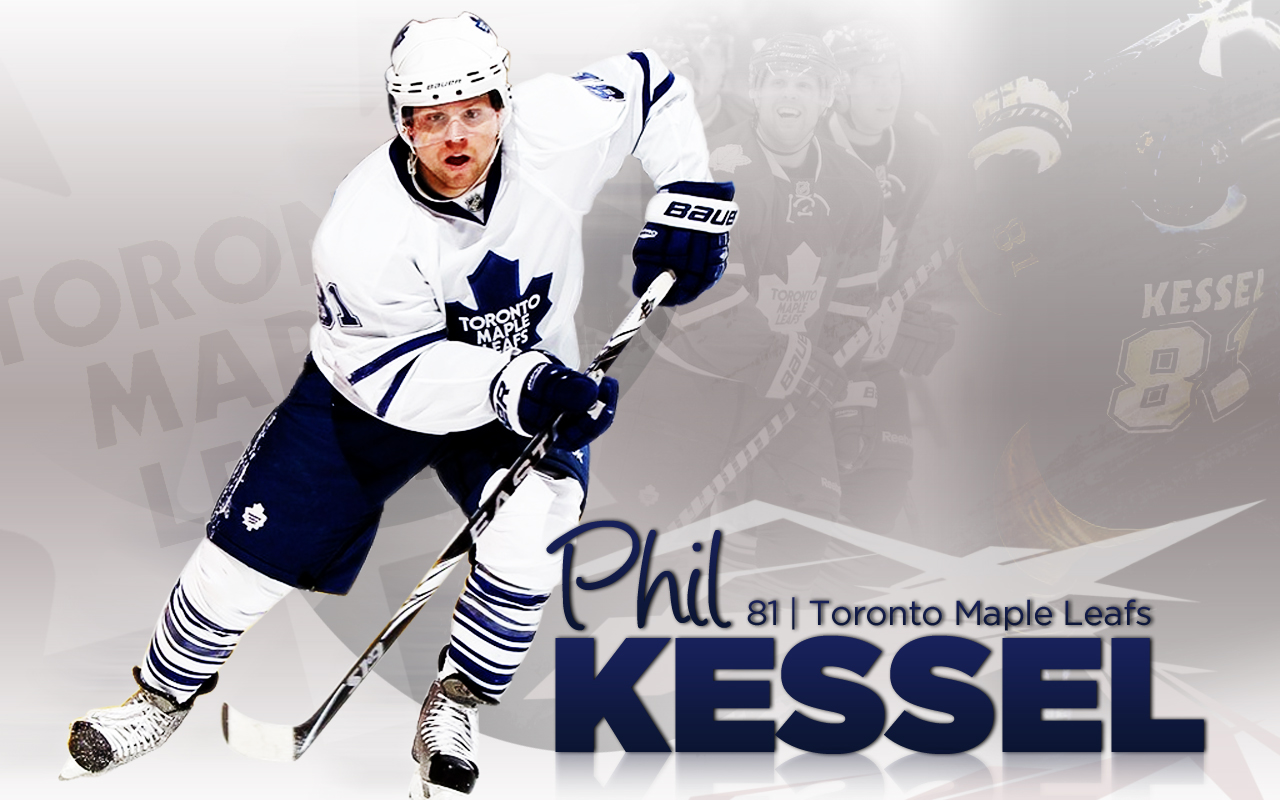The image is a professional advertisement or poster featuring Phil Kessel of the Toronto Maple Leafs. Phil Kessel, number 81, is prominently positioned on the left, looking directly into the camera. He is dressed in the Toronto Maple Leafs' white and blue uniform, which includes a long-sleeved white jersey with a blue Maple Leaf logo on the front, navy padded gloves, navy shorts, white and blue striped socks, and black skates. He also dons a white helmet and holds a black and white hockey stick. Kessel has a ginger beard that adds to his distinctive appearance. The background is a grayish, blurry collage of him and his teammates, adding depth to the image. The text "Phil Kessel, 81, Toronto Maple Leafs" is in blue and located at the bottom right, with "Kessel" standing out prominently. The overall aesthetic is designed to highlight Kessel's dynamic presence, suitable for use as a wallpaper or promotional material.